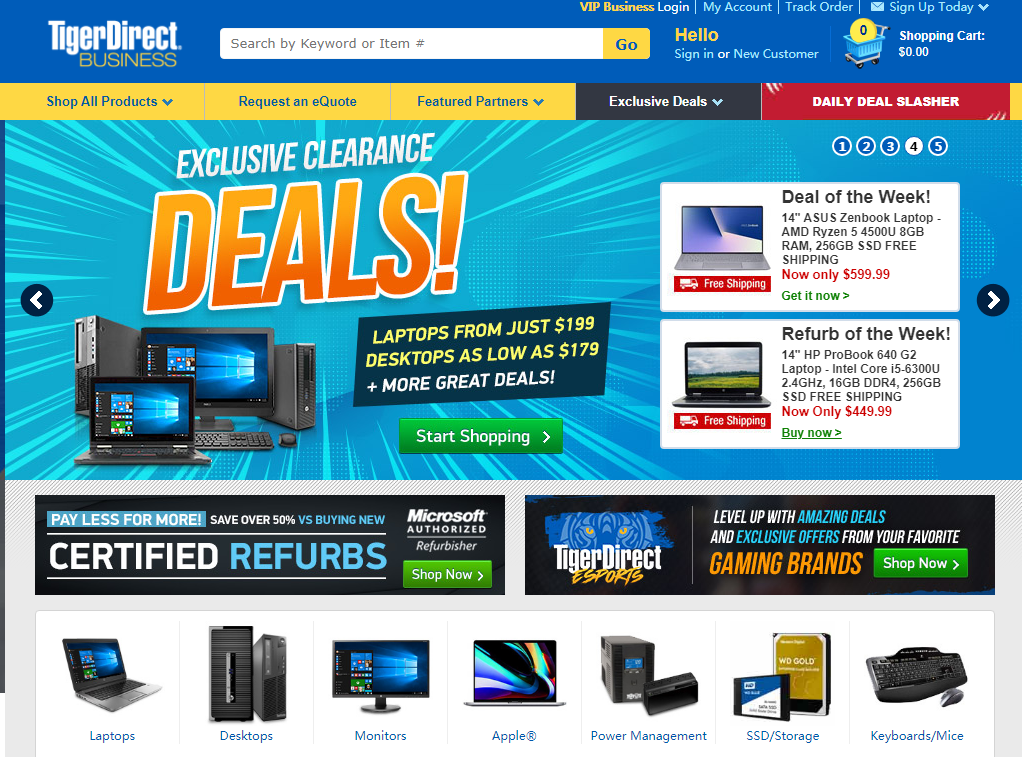The image depicts a detailed close-up of an online clearance deal for computers on the Tiger Direct Business website. The website's logo, "Tiger Direct" is prominently displayed in white text with capitalized "D" and "T" in a single word. Below the logo, the word "Business" is written in thin yellow penmanship.

On the right side, there is a search bar labeled "Search by keyword or item number," accompanied by a "Go" button. Above the search bar, options for "Sign in to VIP," "My Account," "Track Order," and "Sign Up Today" drop-down menus are visible. Additionally, there is an option for new customers labeled "Hello, sign in or new customer" to the right of the search bar, next to a shopping cart icon indicating "0" items.

To the left under the "Tiger Direct" logo, a yellow "Shop All Products" button and a drop-down menu titled "Request a Quote" are visible, offering custom build options through partner collaborations. Exclusive deals are highlighted with a black "Exclusive Deals" button and a red "Daily Deal Slasher" for daily promotional offers.

An ad similar to a newspaper or mail flyer dominates the lower section, headlined "Exclusive Clearance Deals!" in white text. It displays images of tower computers, monitors, and laptops with laptop prices starting at $199 and desktops at $179, both highlighted in yellow. Accompanying this is a "Great Deals" shopping button.

Additional offers include a "Deal of the Week" section and a "Referral of the Week" feature, showcasing two different laptops with their prices and descriptions. Arrows indicate navigation options for viewing up to five different deals. 

Below this are promotions for refurbished products with the slogan "Pay Less for More," and various gaming brands. Categories listed at the bottom include laptops, desktops, monitors, Apple products, power management, storage devices, and keyboards.